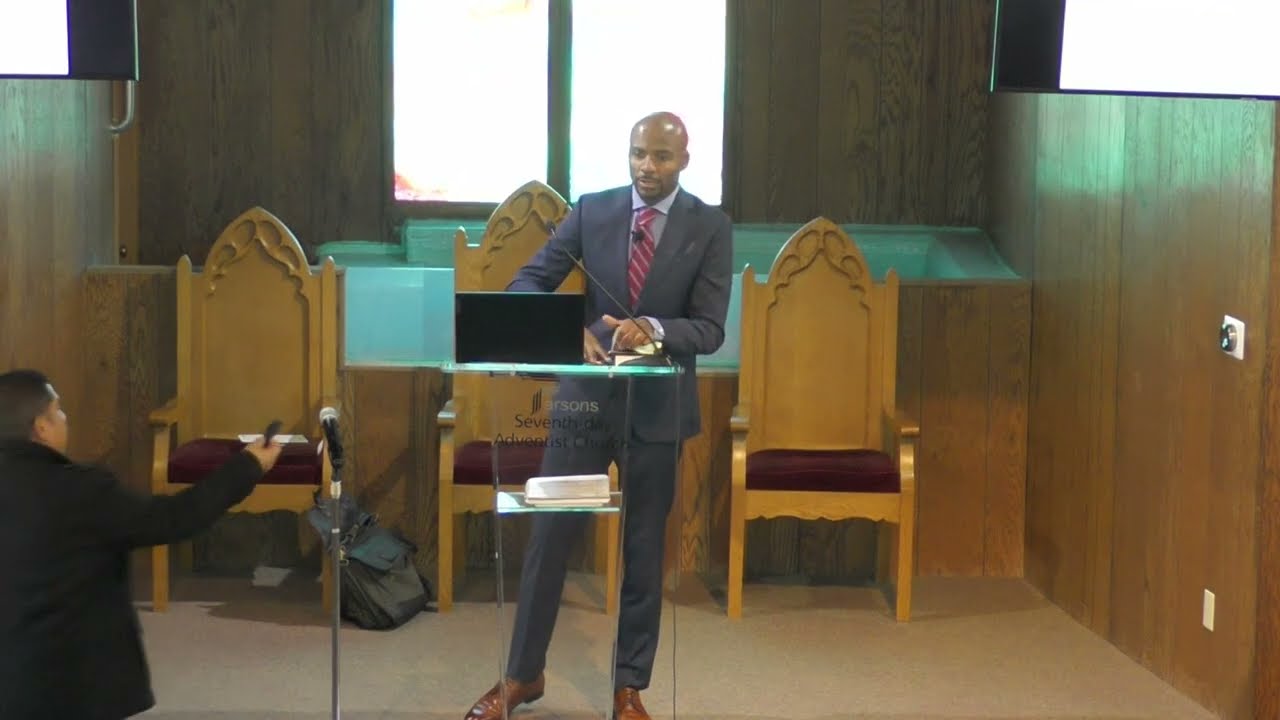A bald, black man stands at the center of the image in front of a glass podium, appearing focused as he looks down and to his left, likely reading from papers he's holding. He is dressed in a gray suit with a blue shirt underneath and a red tie adorned with white stripes, complemented by brown leather dress shoes. The glass podium houses a microphone, suggesting he is speaking at a public event, possibly a press conference or a church sermon. Behind him is a brightly lit window set in a wooden-paneled wall, allowing sunlight to reflect off his head. To the bottom left of the image, a person with short black hair, wearing a black jacket, is partially visible, facing towards the man at the podium. Additionally, the background features three ornate, straight-backed chairs with intricate wooden designs and dark maroon cushions. The room is equipped with a white thermostat control and an electrical outlet on the wall, hinting at a meticulously maintained indoor setting.